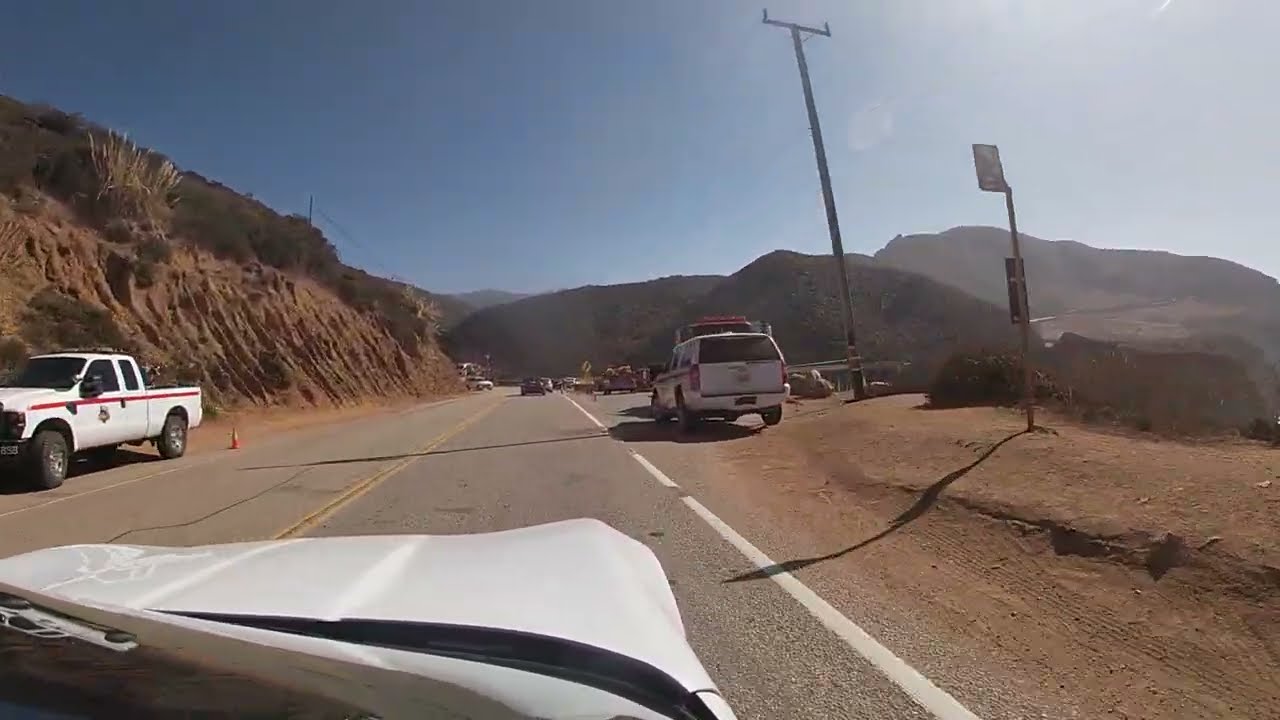This photograph captures a vivid scene from the driver's seat of a white vehicle moving along a picturesque mountain road. The image provides a clear view of the car's front, revealing some markings on the left side of the hood. The paved gray road is lined with yellow center lines and white edge markings. To the left, there's a tall embankment with green bushes and grasses, giving it a rustic appearance. Parked on the roadside are various service vehicles, including a sheriff's car on the left and another white van or truck on the right, both adorned with red stripes and accompanied by traffic cones, likely for an emergency or roadside assistance. Signboards and an electric utility pole are visible on the right side of the road, adding to the detailed roadside scene. Beyond the road, the backdrop features rolling hills under a clear blue sky, bathed in sunlight from the top right corner of the image. The entire scene is framed by natural terrain with no artificial buildings in sight, accentuating the tranquil and scenic mountain environment.